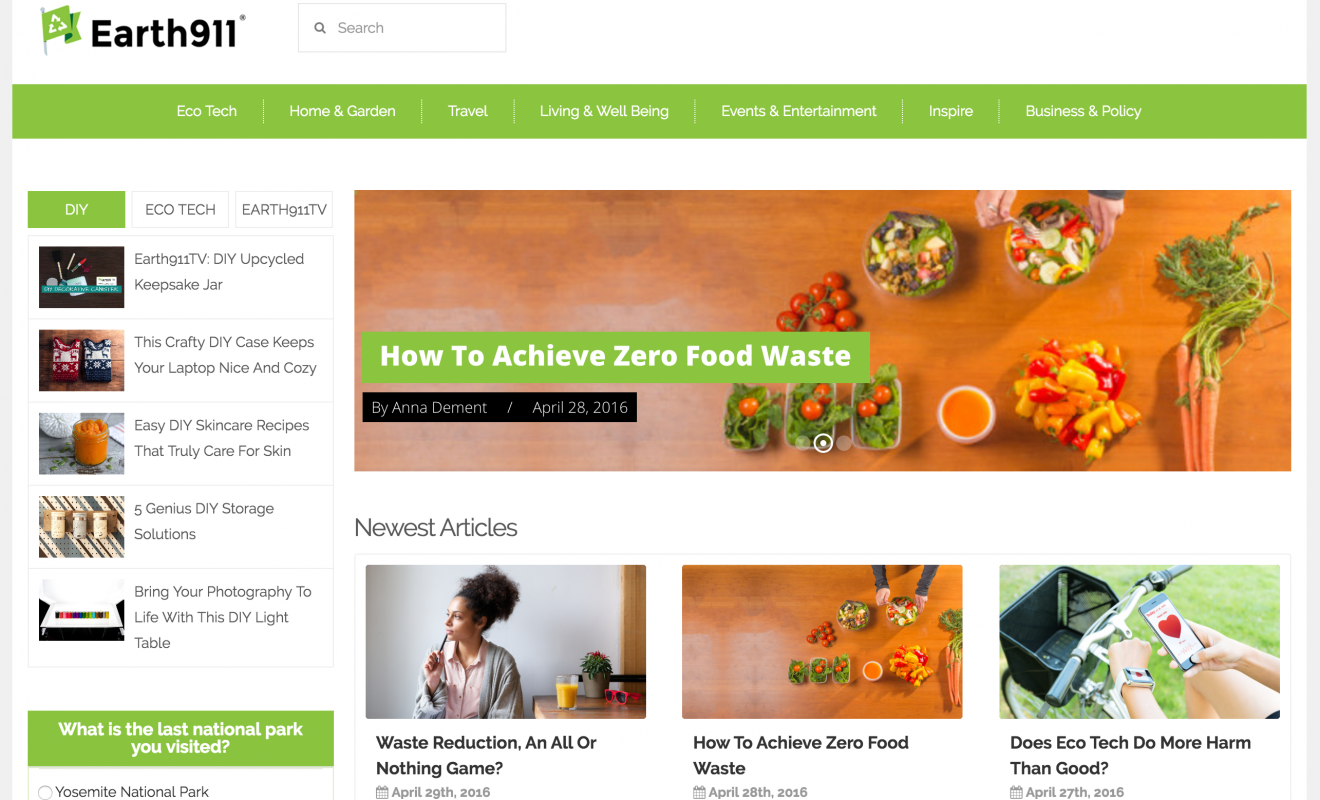On the home page of the Earth911 website, viewed in a desktop format, the design incorporates a predominantly white background accentuated by green elements, reflecting its environmental focus. The top navigation area includes a prominent search bar followed by categories such as Ecotech, Home and Garden, Travel, Living and Well-Being, among others. 

On the left side, there is a section with recent articles, divided into DIY and Ecotech, with DIY currently selected. Featured articles in this section include "Easy DIY Skin Care Recipes" and "Five Genius DIY Storage Solutions." Additionally, there's an article titled "How to Achieve Zero Food Waste" by Anna Demert, dated April 28, 2016, illustrated with a stock photo of food. Below this, there is a list of the newest articles, including thought-provoking titles such as "Waste Reduction: An All or Nothing Game?" and "Does Ecotech Do More Harm Than Good?"